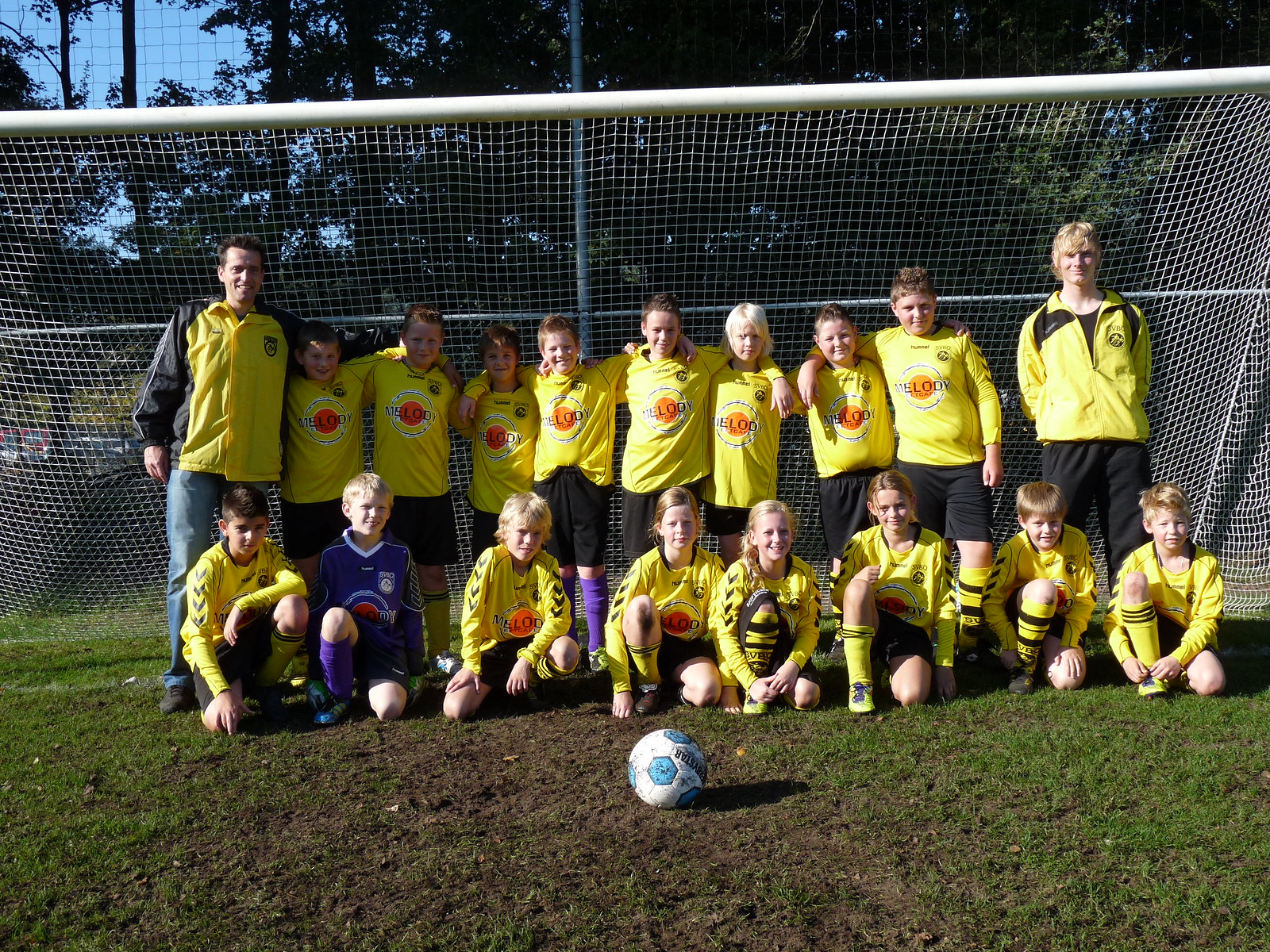This is a detailed team photograph of a youth soccer team, captured on an outdoor grassy field. The image shows two rows of people against a backdrop of a tall chain link fence and closely packed trees, all under an open sky. In the first row, closest to the camera, eight children are kneeling on one knee around a blue and white soccer ball. The second row features another eight children standing with their arms around each other, with two adult coaches flanking them on either side. The children are uniformly dressed in yellow soccer jerseys with black stripes on the sleeves, black shorts, and tall yellow socks, except for one who is the goalie wearing a blue uniform. The coach on the left is in blue jeans and a yellow jacket with black sleeves, while the coach on the right wears similar team colors. A white net of a rectangular soccer goal frames the team, hinting at their unity and team spirit.